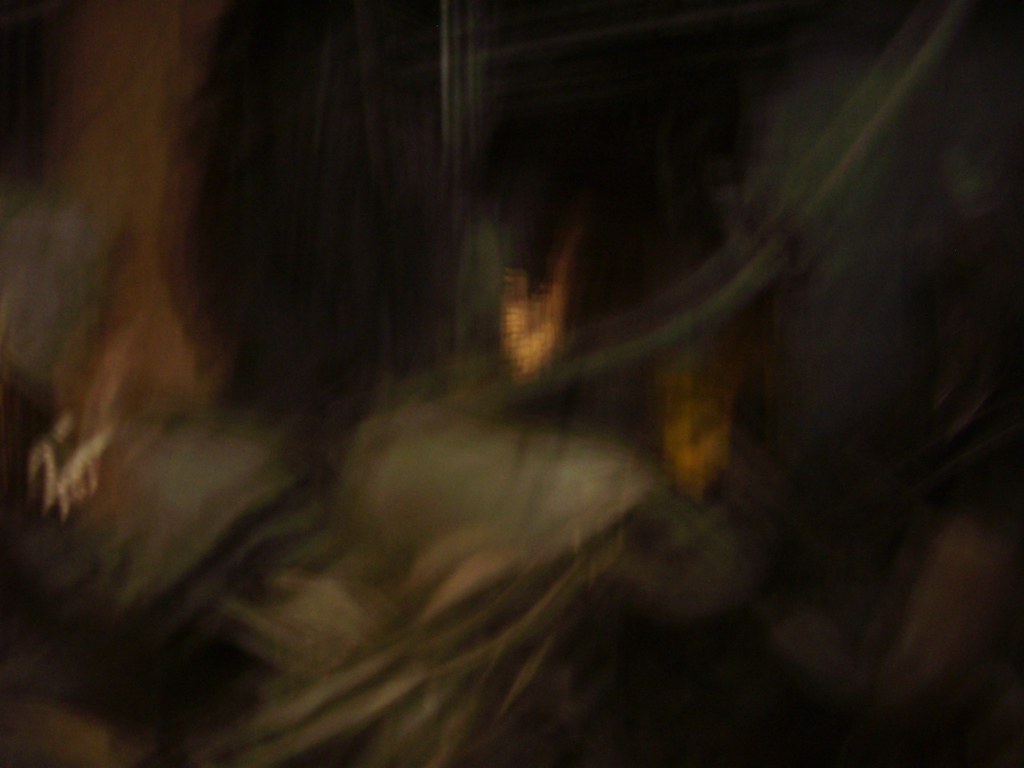This image is an extremely blurry and abstract photograph with a predominantly dark background characterized by deep blacks and heavy shadows. Central to the image are diffused bursts of light in various shades of orange, suggesting fleeting glimpses of fire-like figures, with two starkly prominent orange blurs in the middle and a softer, third glow toward the upper left. Additionally, interspersed grayish-white shadows suggest vague shapes that might interpret as a door or other indistinguishable forms. While some perceive a semblance of a woman draped in green robes, her chest exposed and seemingly engulfed in flames, others suggest abstract patterns akin to a dark Renaissance painting. Threaded with hints of greens, browns, and faint whites, the mysterious and chaotic interplay of colors and motions evoke a sense of potential figures—perhaps people or a solitary arm—amidst an unidentifiable, fiery scene. The entire composition breathes an aura of enigmatic abstraction, capturing the essence of an evocative, albeit hard-to-decipher, artistic vision.